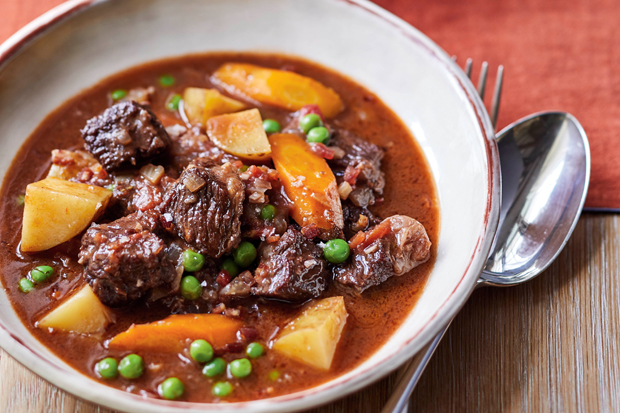This detailed full-color image captures a bowl of hearty stew placed on a white wood tabletop. The light-colored, ceramic bowl features a slightly distressed brown and irregular grayish rim. The stew inside is medium reddish-brown with a hint of oil bubbles on the surface, indicating a rich, thin broth. The stew contains large chunks of browned red meat, likely beef, interspersed with bright green peas and chunks of yellowish potatoes and orange carrots. The bowl is half to two-thirds full, and to the right side, a metallic silver spoon and fork rest on the table, peeking out next to the bowl. The lower part of the image showcases the vertical grain of the wooden tabletop, while the upper part features a soft, suede-like placemat in a rusty red color.